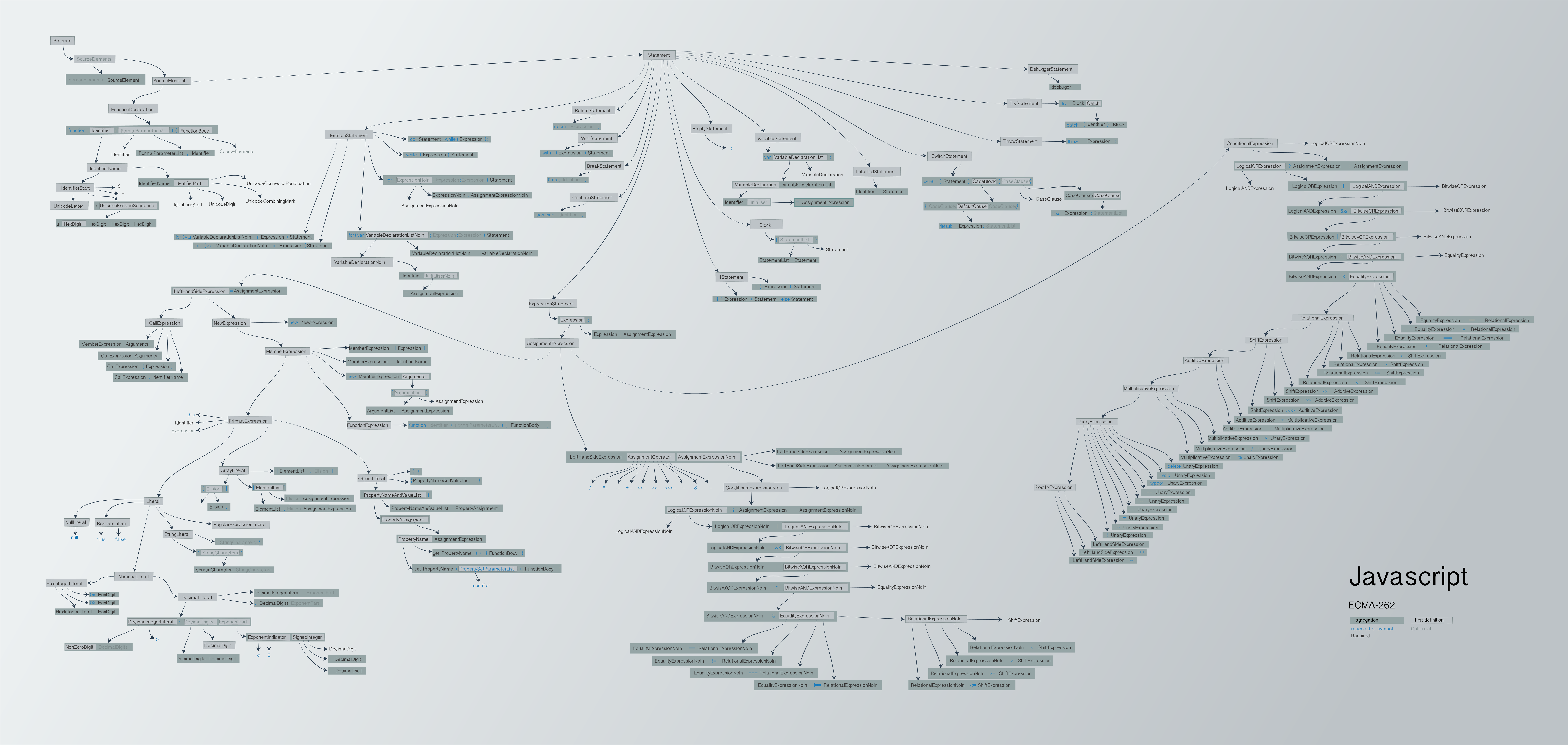This image features a conceptual diagram related to JavaScript, distinguished predominantly by its monochromatic color scheme. Situated in the lower right corner, the term "JavaScript" is prominently displayed with a capital 'J'. Just below this term, a partial string of characters, beginning with "ECM" and followed by three additional, partially obscured characters, is faintly visible.

The entire visual rests on a white background, with text elements presented in black and highlighted in varying shades of gray, ranging from light to very dark gray, approaching black. These highlights create a sense of depth and emphasis on different segments of the text. 

A complex network of thin black lines runs across the page, interconnecting various words. Centrally positioned towards the top of the image, a particular word stands out, serving as a hub with multiple lines radiating outward to other individual words. Additionally, a few other key terms feature several lines extending from them, connecting to other parts of the diagram. Most lines culminate at a single word, but a select few words serve as junctions, branching out to further interconnected terms, adding to the intricacy of the network.